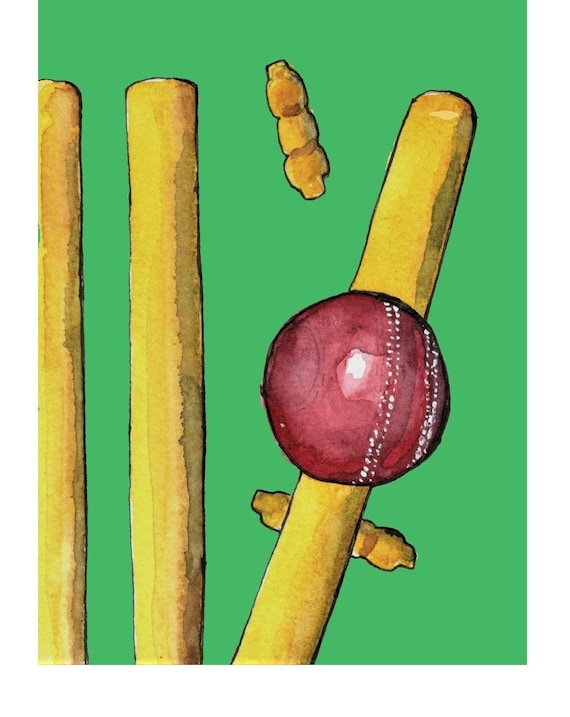The painting features a limish green background with three vertically oriented tan-colored cylindrical objects resembling broom handles or wooden rods. Two of these rods are positioned side by side on the left side of the painting, while the third rod angles slightly from the left upward to the right, positioned on the farthest right. Atop the angled rod sits a shiny, maroon-colored sphere with faint stripes. Surrounding these rods are smaller, segmented oval shapes that have a floating appearance. The overall composition suggests a dynamic scene, possibly reminiscent of abstracted tools from a game like croquet or an assortment of elongated objects and shapes interacting in a whimsical manner.